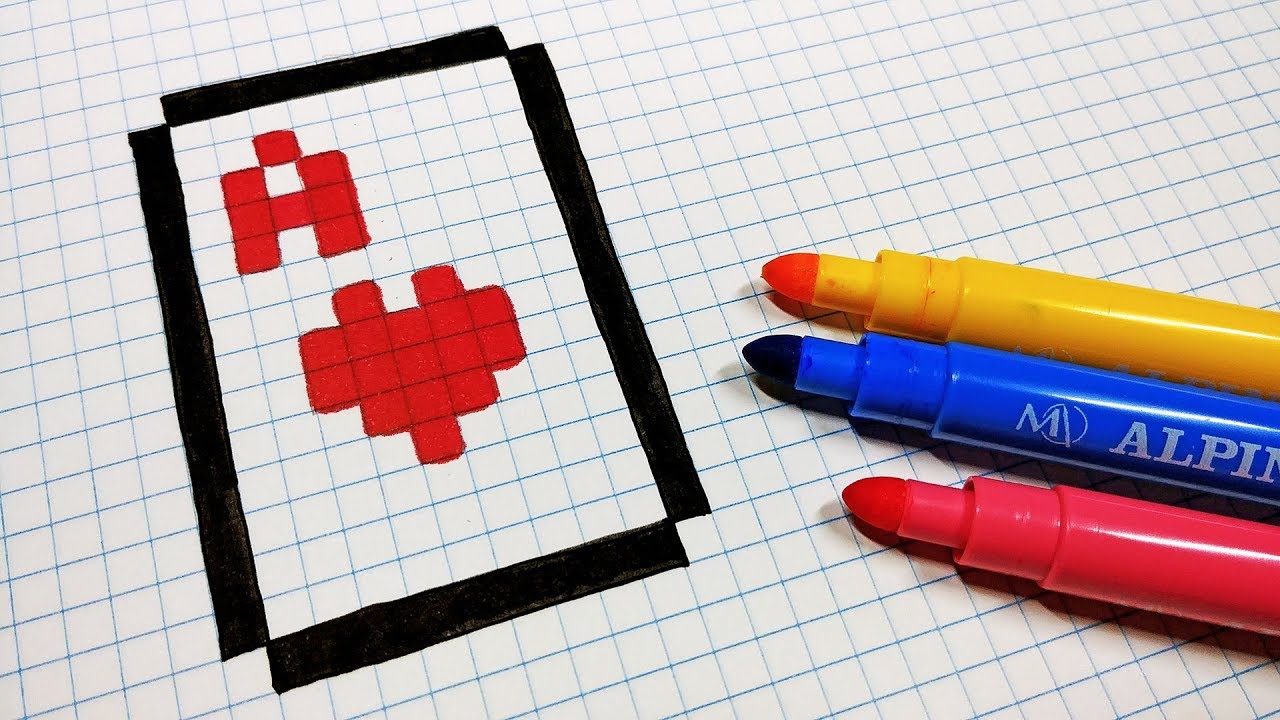In the photograph, a piece of white graph paper with blue lines is prominently displayed, featuring an array of illustrations and markers. The graph paper showcases a tall, black rectangle drawn with a magic marker, with some of its squares filled in red. The four corners of this rectangle remain uncolored, giving it the appearance of an open box. Additionally, in the top left corner of the paper, there is a red, colored-in capital 'A' and a heart. On the right side of the graph paper, three markers are aligned vertically with their tips pointing left. The bottom marker is red, the middle one is blue, and the top one is yellow, although its tip appears more orange. Together, these elements create a detailed and colorful arrangement on the graph paper.